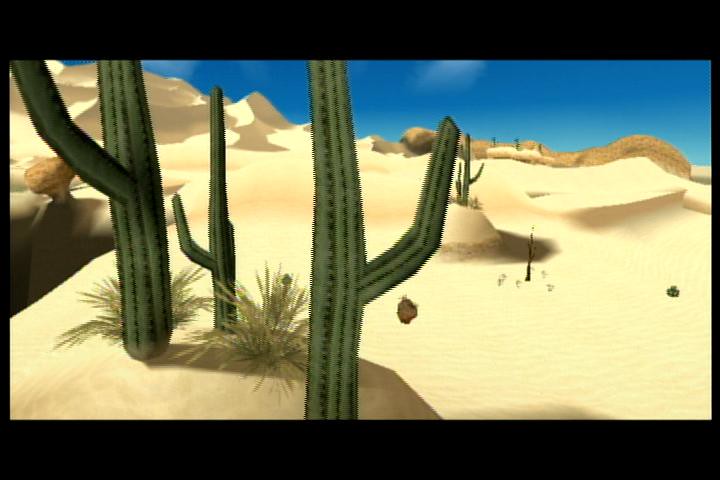A pixelated desert landscape rendered in a video game style, featuring a striking dark blue sky dotted with wispy white clouds. The expansive backdrop is comprised of light tan sandy hills and dunes, accentuated by darker tan shadows that add depth and contrast. The terrain varies, with some areas rising to form mountainous regions. Scattered throughout are large, dark green saguaro cacti adorned with black needles, standing tall and imposing. Complementing the cacti are clusters of light green, spiky bushes, enhancing the rugged and arid aesthetic of the scene. The overall image is characterized by a vibrant, pixelated art style that emphasizes its digital nature.